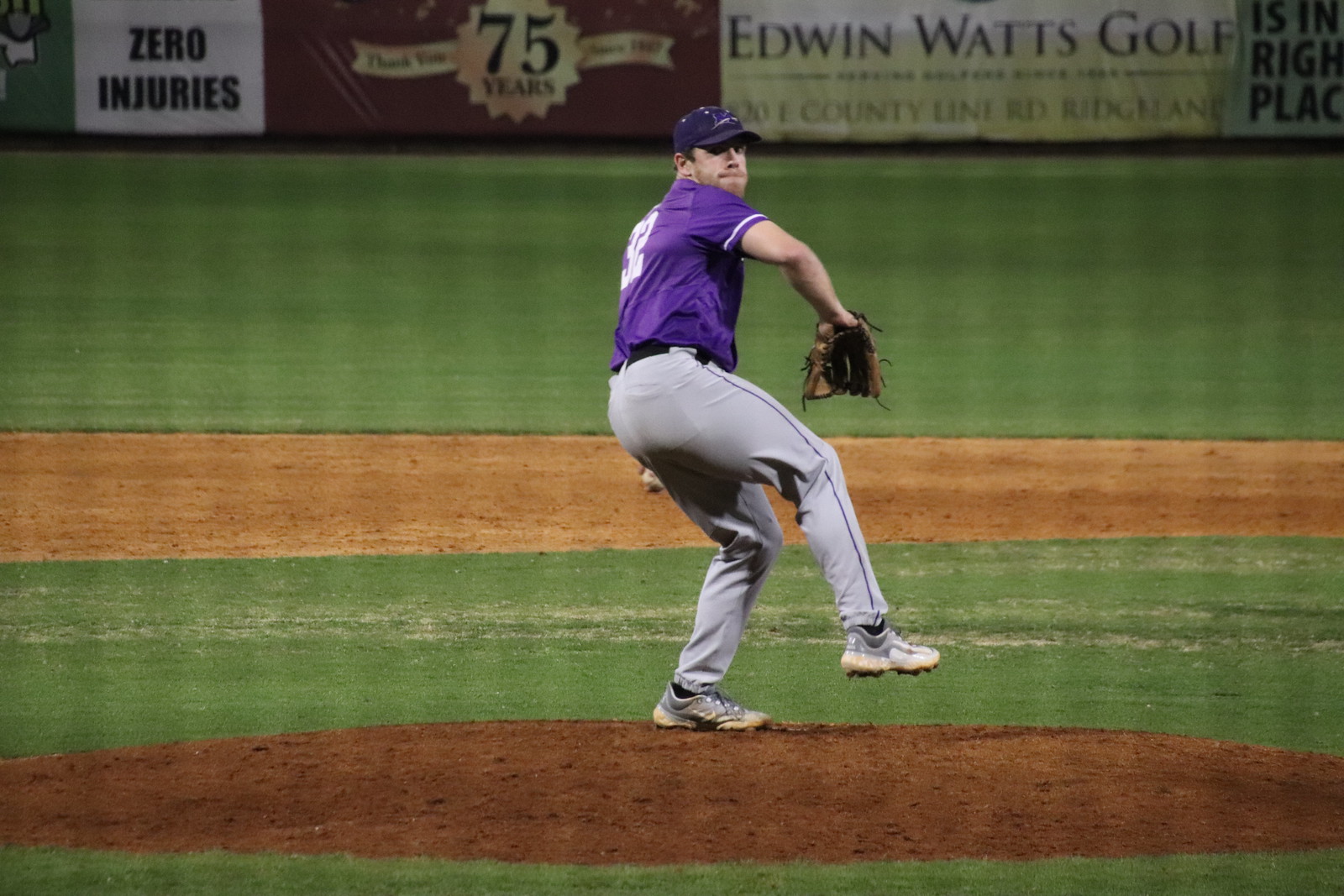This image captures a dynamic moment in a baseball game, focused on a lone pitcher, number 32, who is winding back to throw the ball. The pitcher is prominently positioned at the center of the photograph, standing on the elevated dirt pitcher's mound. He is wearing a purple jersey with white accents, a matching purple cap, light gray pants, and gray shoes. His left hand, which holds the baseball, is poised behind him, while his right hand, donning a brown mitt, is ready for action. The grassy green field stretches out behind him, transitioning from the immediate infield to the more expansive outfield. The wall in the outfield features several advertisements; notably, one reads "zero injuries," another displays a ribbon commemorating "75 years," and there's an "Edwin Watts Golf" sign prominently situated just slightly to the right behind his head. The scene captures a solitary but intense focus on the pitcher's preparation, with no other players present in the frame.